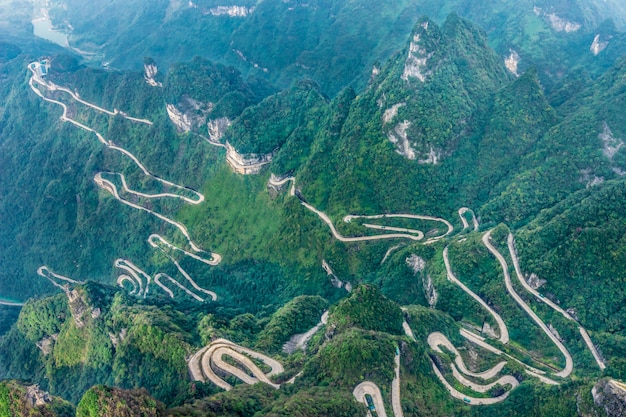This is a captivating overhead aerial photograph of a densely forested mountainside, crisscrossed by an intricate network of zigzagging, winding roads. The lush greenery envelops the jagged, irregular terrain, showcasing a dense canopy of trees interspersed with occasional patches of bare rock. The series of roads, resembling something straight out of a Dr. Seuss book with their insane and crazy design, start in the bottom left corner of the image. They loop and wind repeatedly through the valleys and peaks, creating a labyrinthine path that traverses the entire mountain range. Cars can be seen traveling along these paths, emphasizing their functionality despite their erratic appearance. The road winds up towards the top left, snakes through the middle of the mountains, and eventually loops back down towards the bottom right, before dipping into the dense foliage once more. In the hazy distance beyond the mountains, a lake or river can be faintly discerned in the top left corner, adding a serene backdrop to the complex and verdant scenery.